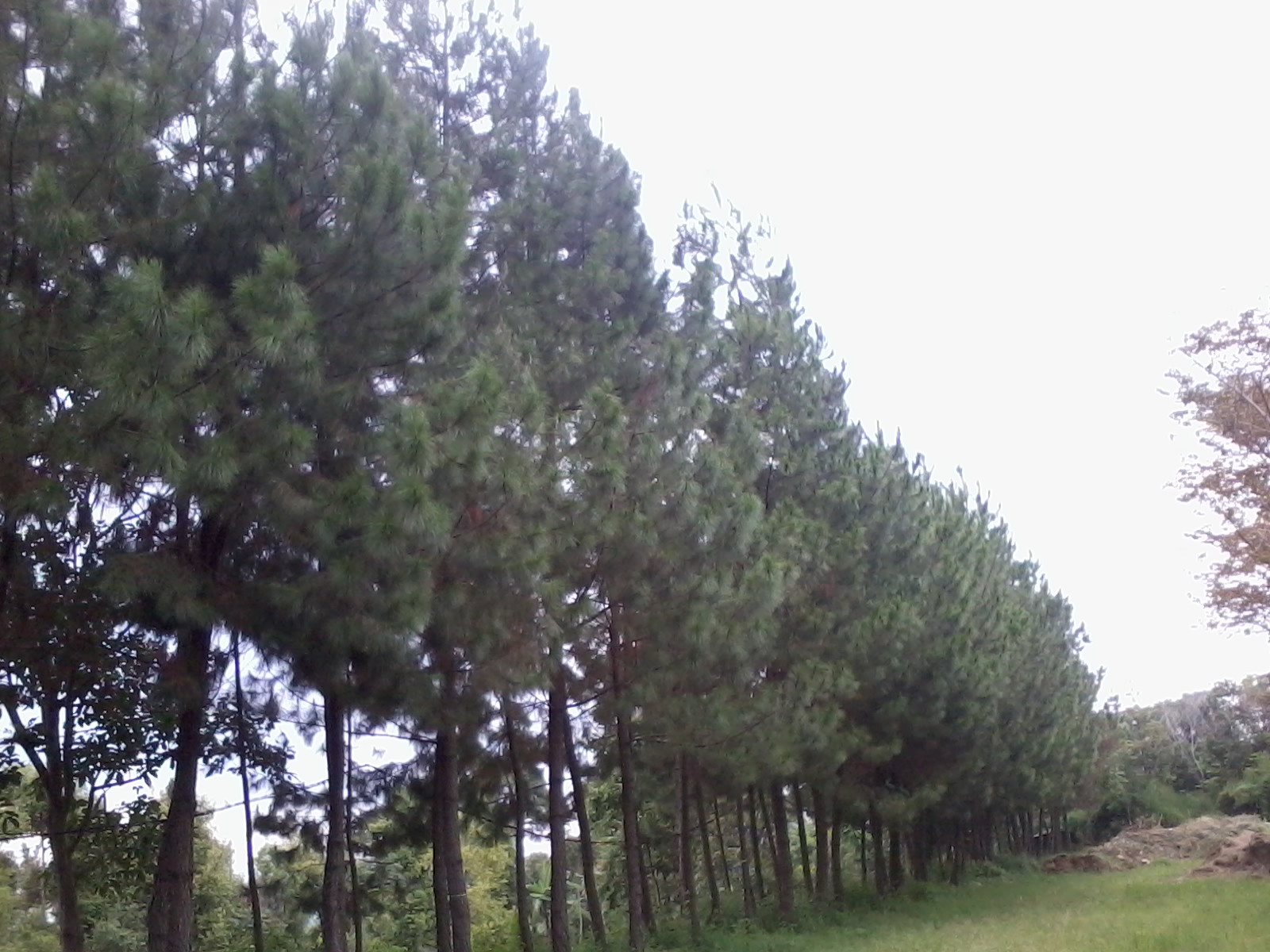This image captures a wide, vertical rectangular photograph of a well-defined border of dark green pine trees that are tall, skinny, and very bushy, creating a dense wall of foliage. These trees stretch from the left edge of the image towards the right, where they gradually recede into the background. Their lower thirds display thin, grayish-brown trunks, transitioning into dense, oval clumps of pine needles above. In the foreground, there's a patch of green grass interspersed with grayish-brown small boulders or rocks. Additionally, towards the background, a little mound of dirt or dead foliage can be seen along with some shorter green trees. The image's upper right corner features a predominantly white, cloudy sky, hinting at a light cloud cover. Notably, a bare, potentially dead tree is faintly visible at the far right edge of the photo, adding a subtle element of contrast to the lush greenery.